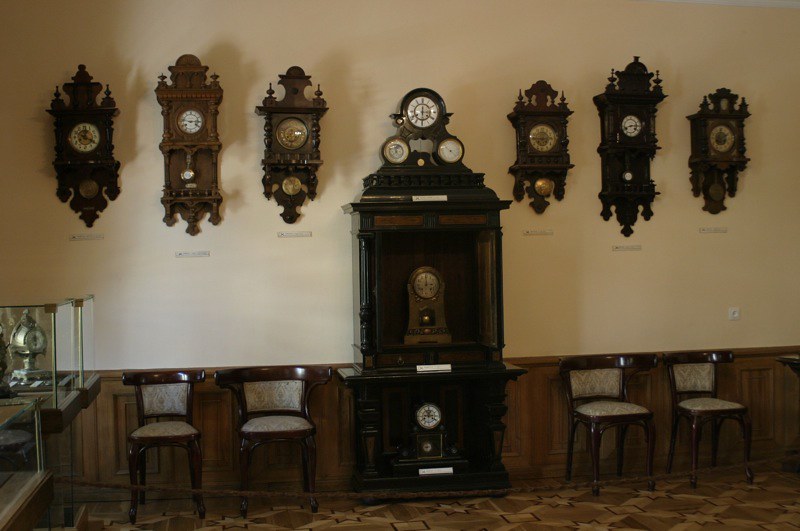The image depicts an antique store filled with an eclectic mix of old-fashioned clocks and furniture. Dominating the center of the scene is a towering grandfather clock, approximately seven feet tall, made of dark, shiny wood with a combination of black and dark brown hues. This ornate clock stands out with its intricate wooden carvings and multiple clock faces. On either side of this central piece, the wall is adorned with six stylishly vintage clocks—three on the left and three on the right. These clocks, resembling cuckoo clocks, feature wooden housings, pendulums, and intricate, pointy wooden designs at the top.

To the left of the grandfather clock, there's a metallic clock showcased in a glass display case, suggesting a sales kiosk area typical of an antique store. Below and around the clocks, there are four old-fashioned wooden chairs with fabric seats; two of these chairs have brown frames with white cushions and are positioned prominently on the left and right sides. Additionally, the floor features a crisscross wooden pattern that adds a rustic charm to the setting. The intricate details and layout of the clocks, along with the classic furniture, emphasize the store's nostalgic and historical ambiance.